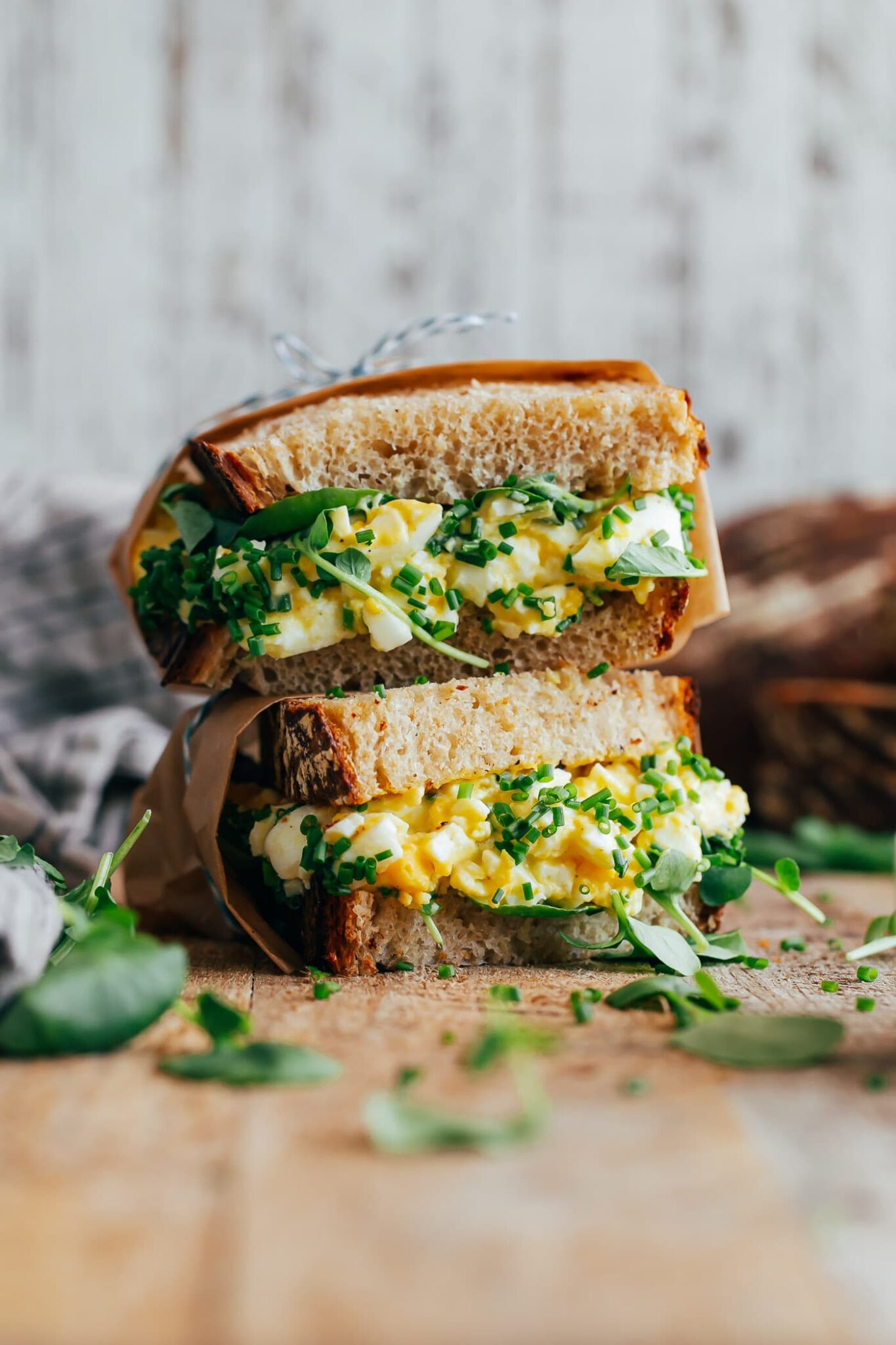The photograph showcases an egg salad sandwich, captured at a close angle as if the camera were placed directly on the wooden countertop where the sandwich rests. The sandwich is presented in two neatly cut halves, suggesting that a single sandwich has been sliced for easier consumption. Both halves are wrapped in paper, adding a rustic touch. The bread is crisply trimmed, holding together a creamy mixture that likely includes cooked eggs, finely chopped green onions, and possibly mustard, giving it a yellowish hue. Scattered across the wooden surface in the foreground are small, vibrant green leaves, adding a fresh, decorative element. The background remains out of focus, featuring indistinct objects, thus drawing attention squarely to the sandwich itself.